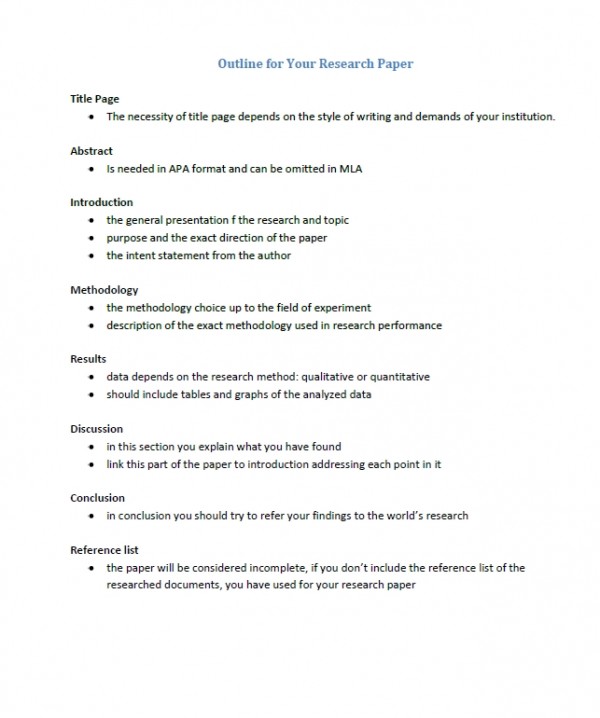The image depicts a printed handout titled "Outline for Your Research Paper" displayed in blue fonts at the top center of a white background. The detailed outline, formatted with bullet points, begins with “Title Page,” which emphasizes that the necessity of a title page depends on the writing style and the requirements of the institution. Next, “Abstract” indicates that it is necessary for APA format and can be omitted in MLA. 

The “Introduction” section is then outlined with points about the general presentation of the research and topic, the purpose and exact direction of the paper, and the intent statement from the author. Following this is “Methodology,” which covers the choice of methodology depending on the field of experiment and a detailed description of the exact methods used in the research.

The “Results” section mentions that the data presented depends on whether the research is qualitative or quantitative and should include tables and graphs of the analyzed data. In the “Discussion” section, it is advised to explain the findings and link this part of the paper to the introduction by addressing each point previously mentioned. The “Conclusion” suggests referring the findings to the broader context of existing research. Lastly, the “Reference List” is noted as crucial, stating that the paper will be considered incomplete without the references of the sources used.